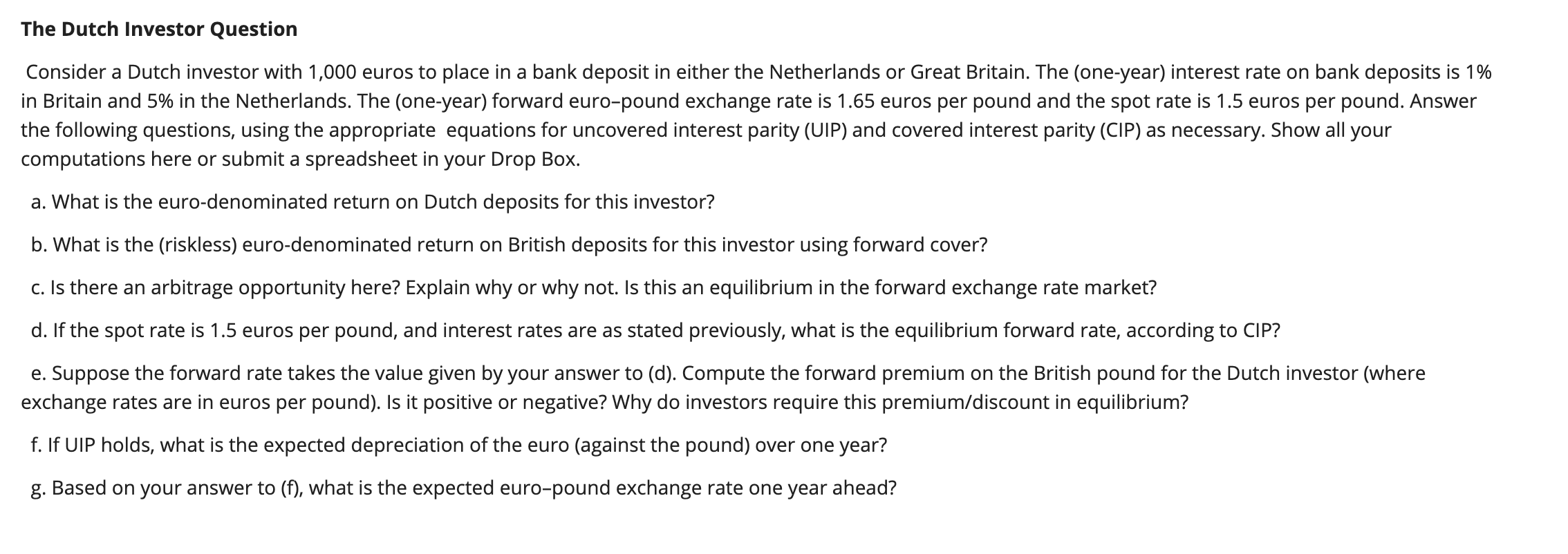The image features a detailed financial problem set prominently situated on the top left-hand corner in bolded black text. It begins with the heading "The Dutch Investor Question" and contains a paragraph following this introductory line. The paragraph reads:

> _"Consider a Dutch investor with 1000 euros to place in a bank deposit in either the Netherlands or Great Britain. The one-year interest rate on bank deposits is 1% in Great Britain and 5% in the Netherlands. The one-year forward euro-pound exchange rate is 1.65 euros per pound, and the spot rate is 1.5 euros per pound. Answer the following questions using the appropriate equations for uncovered interest parity (UIP) and covered interest parity (CIP). As necessary, show all your computations here or submit a striped sheet in your Dropbox."_

Below this paragraph and positioned in the middle left of the image, there is a list of questions labeled from A to G, each accompanied by its own line. For instance:
- **A**: "What is the euro-denominated return on Dutch deposits for this investor?"
- **B**: "What is the riskless euro-denominated return on British deposits for this investor using forward cover?"

This pattern continues with questions outlined for each subsequent letter down to **G**.

The image appears to be a comprehensive problem set aimed at understanding the practical application of financial concepts such as uncovered interest parity (UIP) and covered interest parity (CIP).